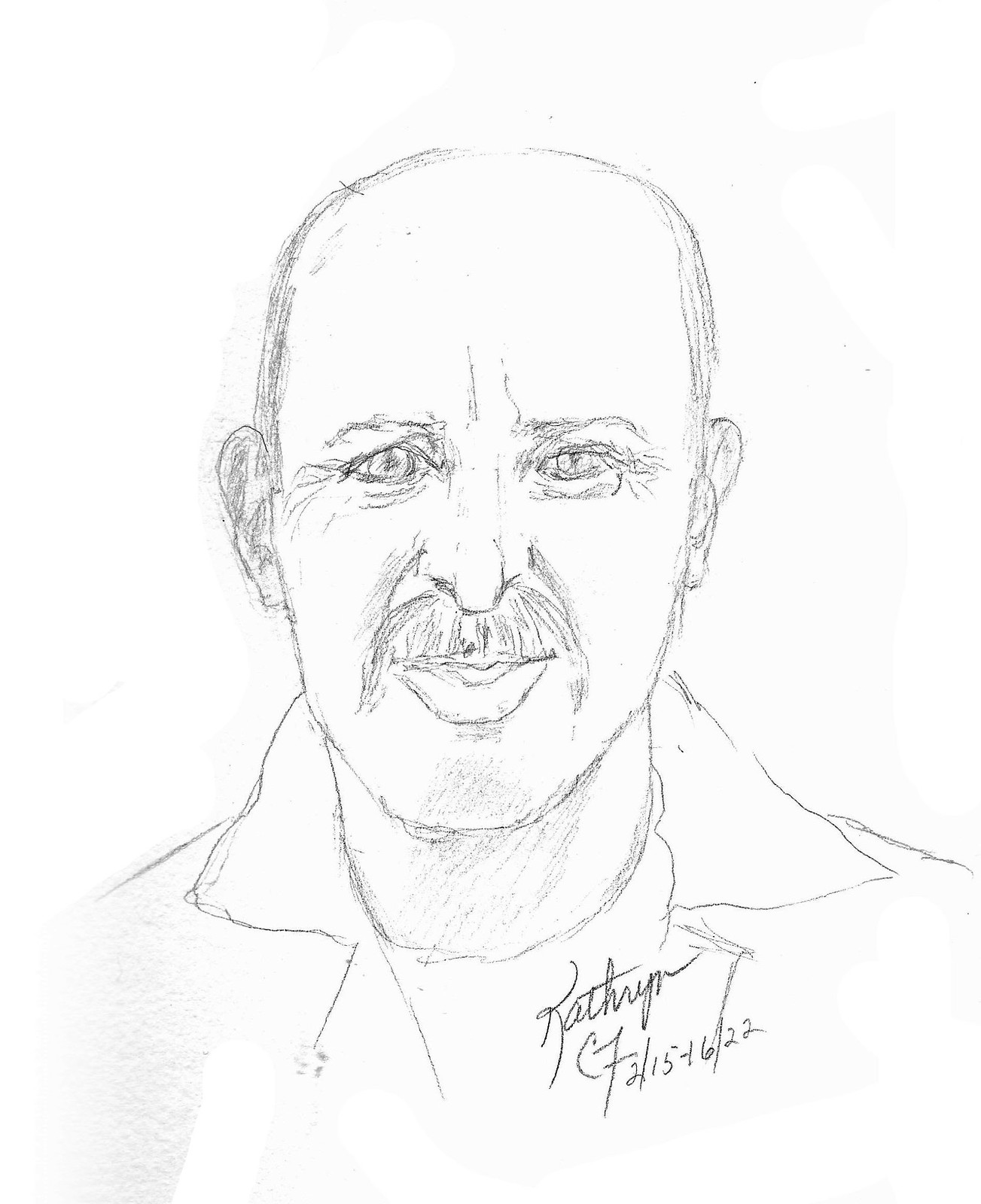This is a detailed pencil sketch of a middle-aged bald man with a mustache, showcasing his face and shoulders in a bust-style portrait. The man, who appears to be in his 40s or 50s, has subtle signs of aging such as crow's feet around his eyes. He is dressed in a collared coat over a white undershirt, with a naturally composed expression that includes a slight smile. The sketch reveals a moderate amount of shading and detail, enough to allow for the person’s identification, yet it has an amateur quality with a simple outline on a white background. The artist, Catherine C.F., has signed the piece below the man's neckline, and it includes the dates 2/15/22 and 2/16/22, suggesting it was created over these two consecutive days. There is no information about the identity of the man, leaving it ambiguous whether he is a family member, friend, or simply a subject. The overall feel of the drawing is akin to a police sketch but rendered with more warmth and personal touch, devoid of any sinister undertones.